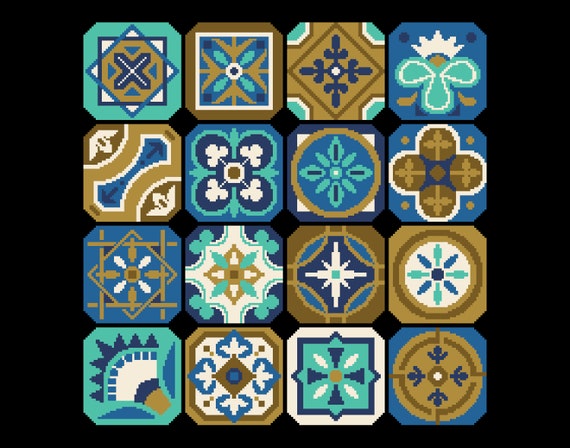This digital image showcases a 4x4 grid of 16 unique tiles, each featuring a different geometric pattern with smooth, pixel-art-like designs. The tiles, which have their corners cut off to form an almost-square shape, are set against a contrasting black background. With a consistent color palette dominated by shades of blue, turquoise, brown, and taupe, these tiles exhibit a refined pixelated look that recalls computer game aesthetics. Intricate geometric shapes like squares, circles, ovals, and notably, multiple forms of crosses or Xs are prevalent, exemplified by the top-left tile which features an X bordered in light blue, overlaid with intersecting squares and a diamond. The artwork contains no text, signatures, or copyright symbols, allowing the focus to remain on the sophisticated interplay of colors and shapes within each tile.